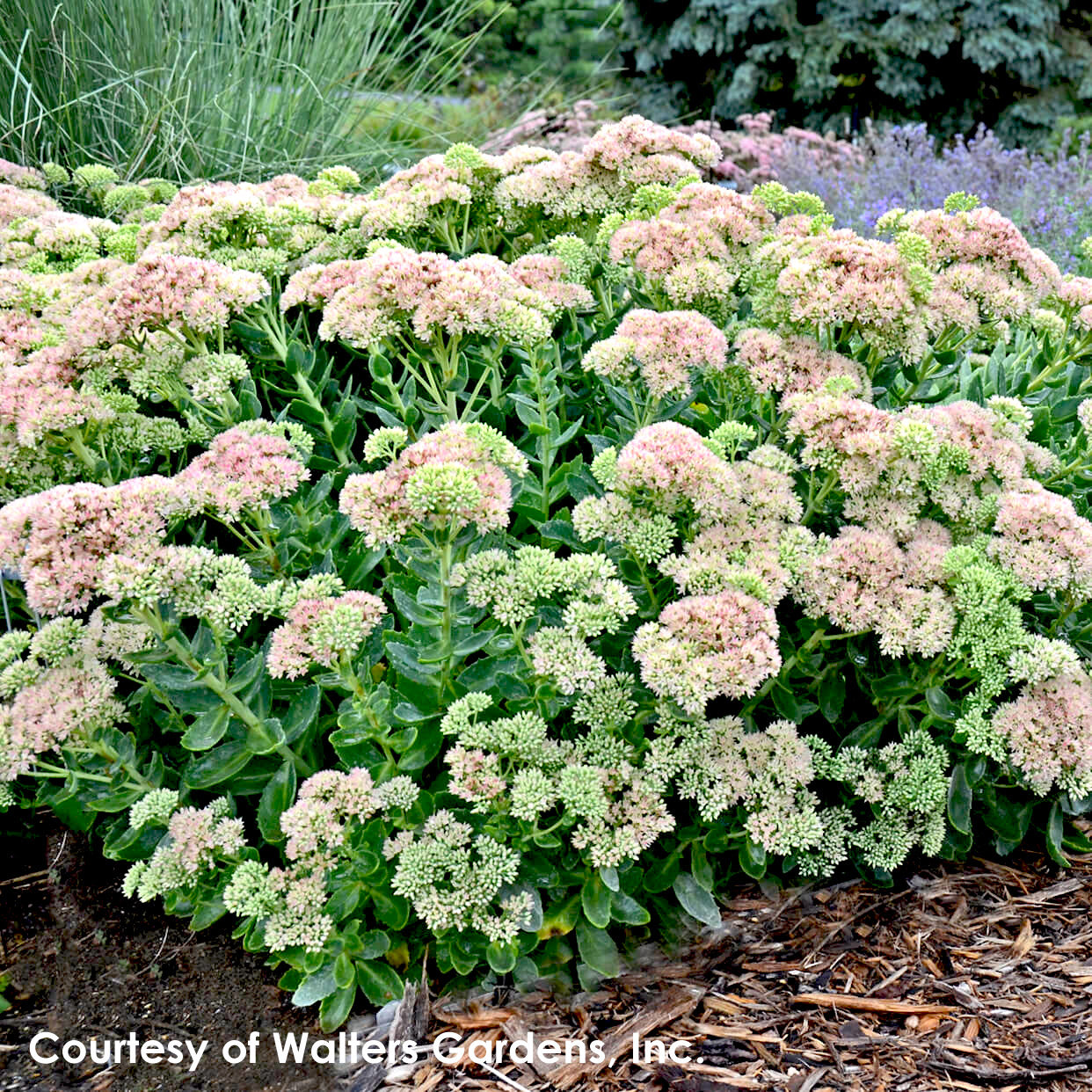The image captures an outdoor garden scene focused on a prominent bush of Autumn Joy Sedum flowers, identifiable as Sedum telephium. The bush comprises flowers that transition from green buds to light pink blooms, arranged in dense, hydrangea-like clusters. These clusters sit atop long stalks with thick, large leaves. The bush is situated in an area with woodchip ground cover. In the background, the top left of the image features tall green grasses, while the top right side showcases a cluster of small, light purple flowers, likely lavender. The entire scene is accompanied by a white text at the bottom of the image that attributes the photo to Walters Gardens Incorporated.